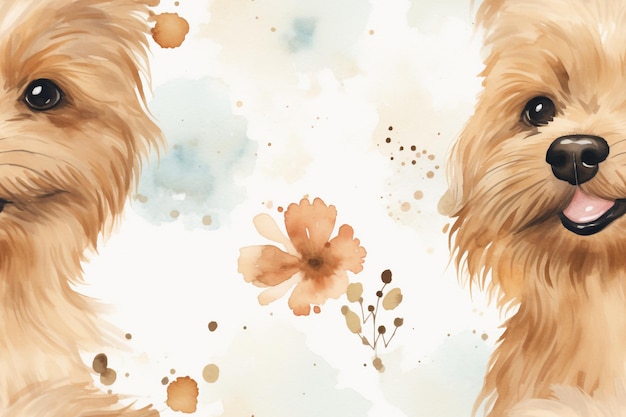This artwork presents a playful watercolor drawing of two small, shaggy beige and brown dogs, potentially terriers, set against a predominantly white background. On the left side, the dog's face is partially visible, showing its left eye, half of its mouth with a black outline, and white whiskers. On the right side, another dog of similar colors is depicted more fully: its black button nose, open mouth with a small tongue peeking out, black-outlined lips, and shaded chin give the impression of a little beard. Both dogs have expressive dark eyes and floppy ears.

Between the dogs are muted pink flowers, small unbloomed flower stems, and blue splotches, which add a delicate contrast to the otherwise serene background. There are also pale blue and pink shaded clouds interspersed, giving the overall artwork a whimsical, wallpaper-like appearance.